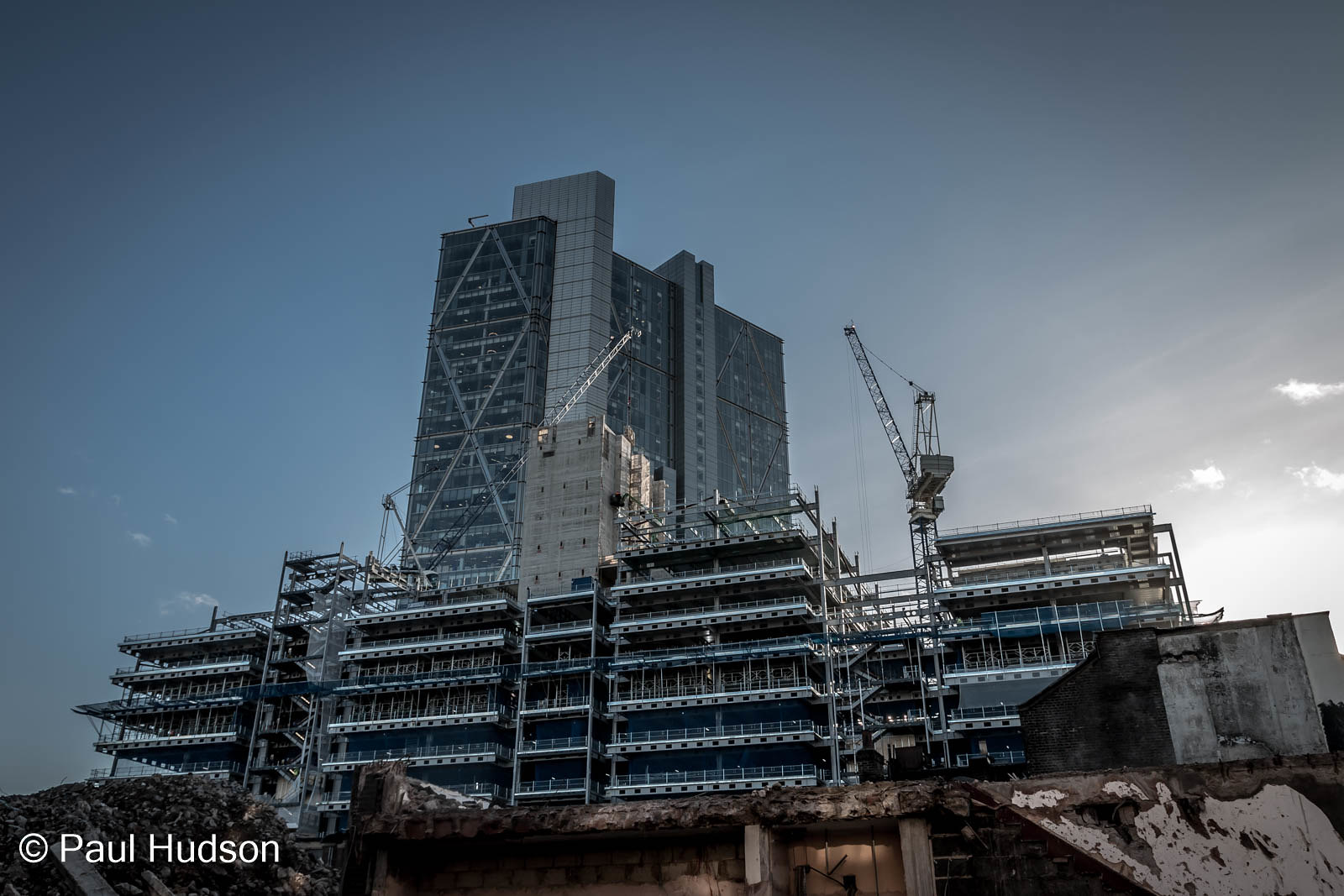The photograph captures a bustling high-rise construction site against the backdrop of a partially cloudy blue sky, with the brightness of the sun peeking in from the bottom right corner. The primary focus is on the major building being built, which has already progressed up to several stories, estimated to be around seven floors. The structure showcases exposed girders, beams, and a central cement-enclosed elevator shaft, indicating its potential to reach several more stories higher. Two towering sky cranes—one positioned on the right side and another towards the left center—dominate the scene, tirelessly hoisting materials. In the background stands a completed gray and black skyscraper featuring a distinctive diamond-shaped design across its facade, contrasted by taller white sections. This completed building, possibly an office or hotel, adds depth to the scene. The foreground reveals a rocky terrain, adding a raw, industrial feel to the photograph, which is attributed to photographer Paul Hudson, as noted by the copyright mark in the lower left-hand corner.